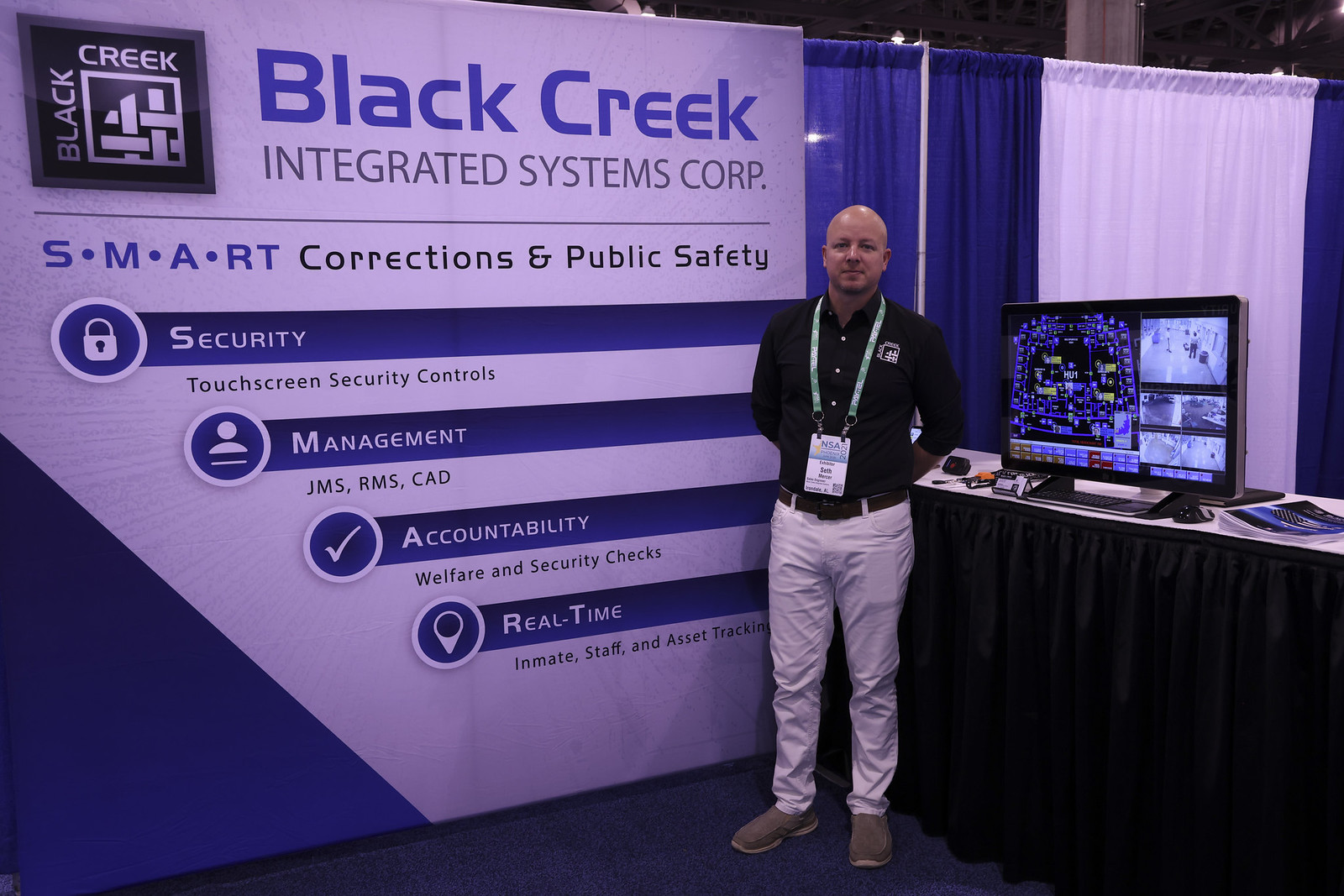At a marketing convention booth, a bald white man wearing a black shirt, green lanyard, white pants, and gray shoes stands prominently. To his left is a short table draped in black with a white tablecloth, on which sits a square flat-screen TV displaying various video camera feeds. He is positioned in front of a large advertising sign featuring blue and gray text. The top of the sign reads "Black Creek" in blue, followed by "Integrated Systems Corp" in gray. To the left, the sign displays in blue text “S • M • A • RT,” and further below in black text, it reads "corrections and public safety." The background alternates between blue and white curtains, enhancing the professional setting.